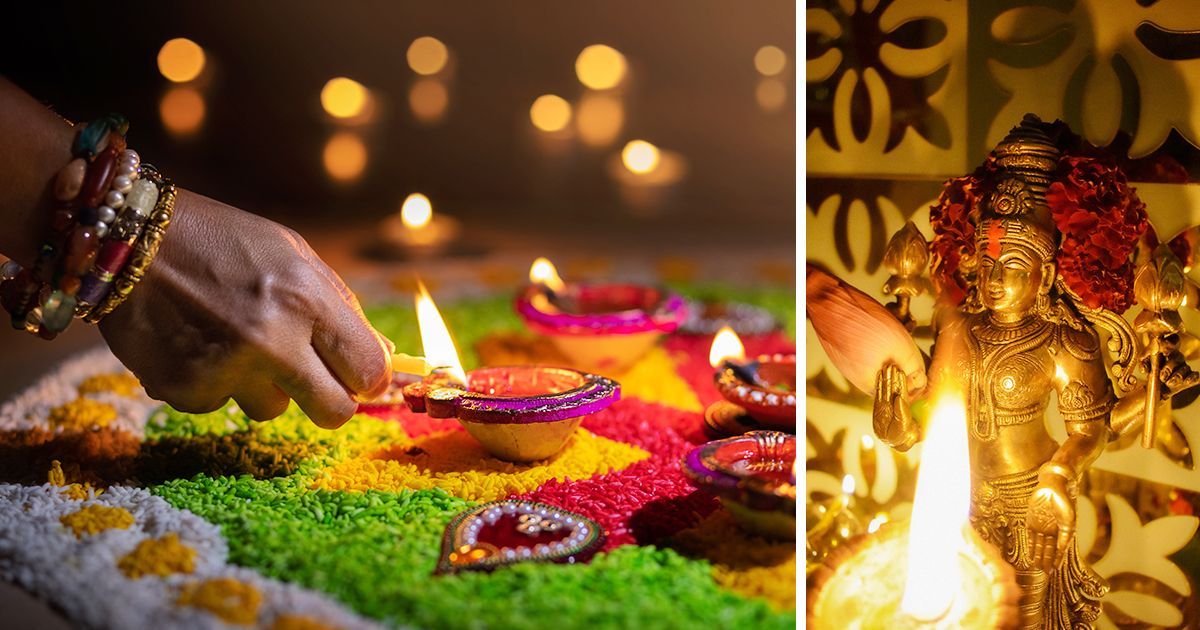This split-image composition features two distinct yet connected scenes. On the left, a person’s hand adorned with several colorful bracelets—pearl, burgundy, purple, gold, and green—holds a match and lights a vibrant cake. The cake itself is a kaleidoscope of pink, yellow, green, and white colors, resting on a colorful mat with a floral pattern featuring red, yellow, green, and white accents. This intricate mat adds to the celebratory and festive atmosphere. 

To the right, a gold statue exudes an Egyptian or Hindu religious aura, distinguished by its elaborate armor and large helmet. In front of this statue, a candle with a bright, large flame burns, casting a warm glow. The combination of the candle flame and the gold statue imbues a sense of reverence and sacredness to the scene, possibly indicating a ceremonial event. The juxtaposition of the hand lighting the festive cake and the solemn, glowing statue suggests a blend of celebration and spirituality, portraying a rich, multi-faceted cultural moment.